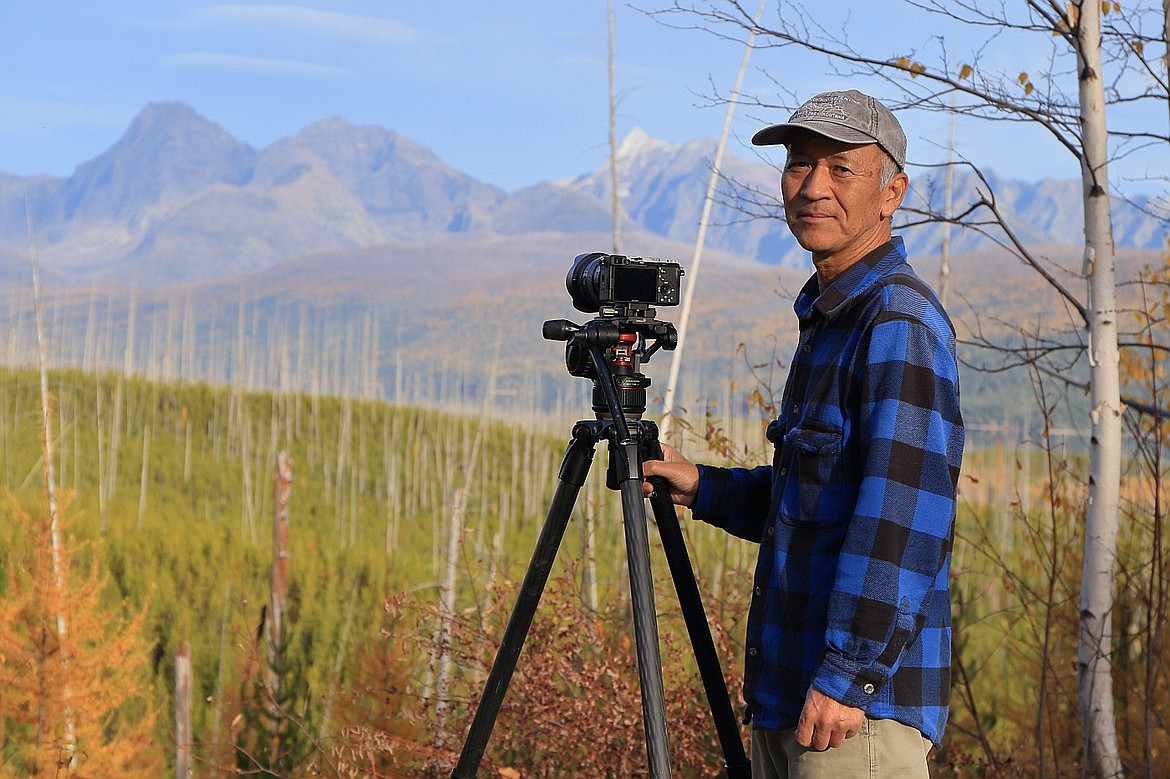The photograph captures a serene outdoor scene featuring an older Asian male photographer, likely in his 40s to 60s, standing on the right side of the horizontal frame. He is wearing a grey baseball cap, a blue and black plaid flannel shirt, and tan khaki pants. The man, tanned and looking at the camera with a gentle Mona Lisa smile, rests his right hand on a large black camera positioned on a tripod at the center of the image. 

The backdrop reveals a picturesque landscape, with a grassy hill leading up to distant rocky mountains, one of which is snow-capped. The sky is a clear blue, adorned with faint, wispy clouds. Flanking the photographer on his right is a slender white sapling with bare branches, some holding a few dead leaves. The foreground features patches of tall grasses and some reddish-white bushes, indicating an autumnal setting. The overall ambiance is one of tranquil natural beauty, captured through the lens of an experienced photographer.